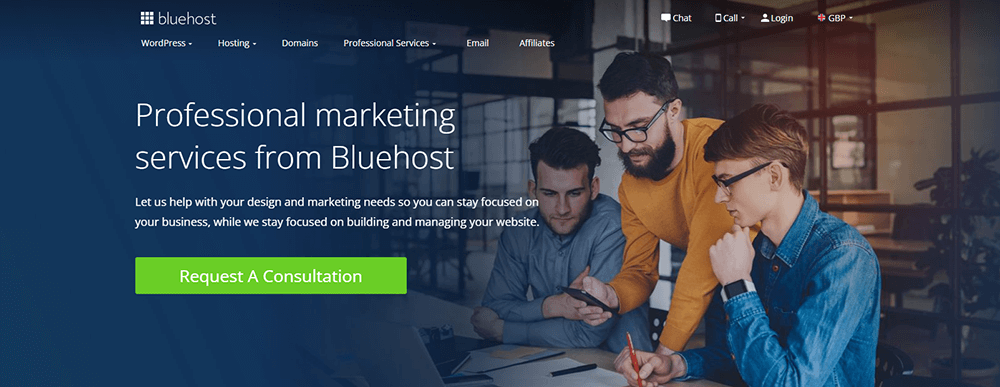The image showcases a large rectangular webpage viewed in landscape orientation, divided into two main sections. The left side of the webpage has a dark blue hue and prominently features white text stating "Professional Marketing Services from Bluehost." Below this text, there's a green rectangular button labeled "Request a Consultation."

On the right side of the webpage, there's a photo depicting three men working together. The man in the middle is standing and leaning over a desk, holding a black rectangular smartphone in his right hand. He has a bushy brown beard, short brown hair, and is wearing black-framed eyeglasses and an orange long-sleeved shirt. Flanking him are two seated men who are both looking at the smartphone. The man on the left has short brown hair and pale white skin, while the man on the right, who also has short brown hair and black-framed eyeglasses, is wearing a blue denim jacket and a black square watch on his wrist.

At the top right corner of the webpage, there are buttons for "Chat," "Call," "Login," and "Language." On the top left, under the Bluehost brand name and logo, there are navigational buttons for different sections such as "WordPress," "Hosting," and "Domains."